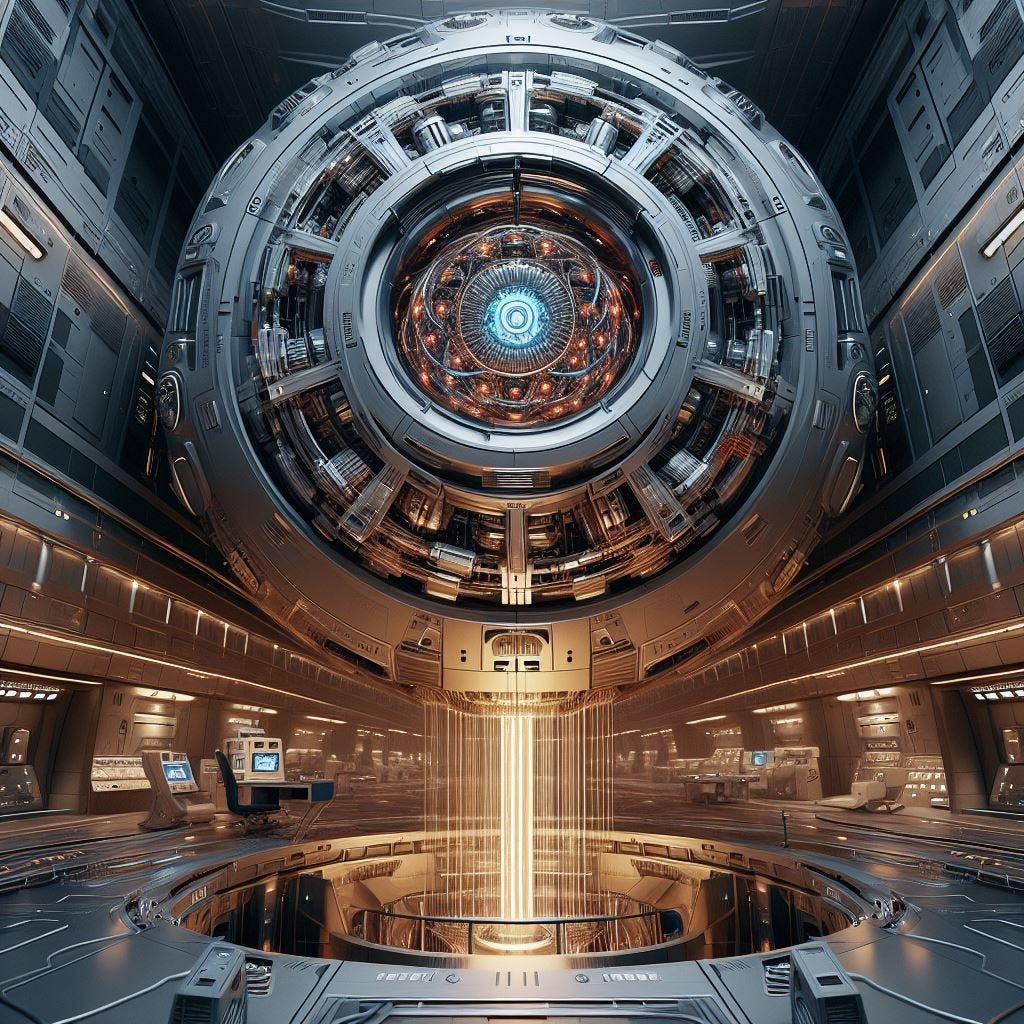The image depicts the interior of a futuristic spaceship, focusing on a deck dominated by a massive, circular reactor core situated in the top center. The reactor core, resembling stereotypical sci-fi warp cores from movies and novels, occupies about two-thirds of the image. It emits a bright beam of light downward, suggesting it is the reactor in operation. The core's surface is characterized by an intricate design, featuring a central "eye" with a blue light surrounded by a circular pattern. Surrounding this core is a depression area filled with various terminals and control panels, indicating this is a critical area of the ship. The overall color scheme is metallic, predominantly silver and grey, complemented by a soft orange glow emanating from the core. The scenery hints at a multi-level structure, with lower levels housing computer equipment and the upper stories featuring hallways that wrap around the core, adding depth and complexity to the environment.